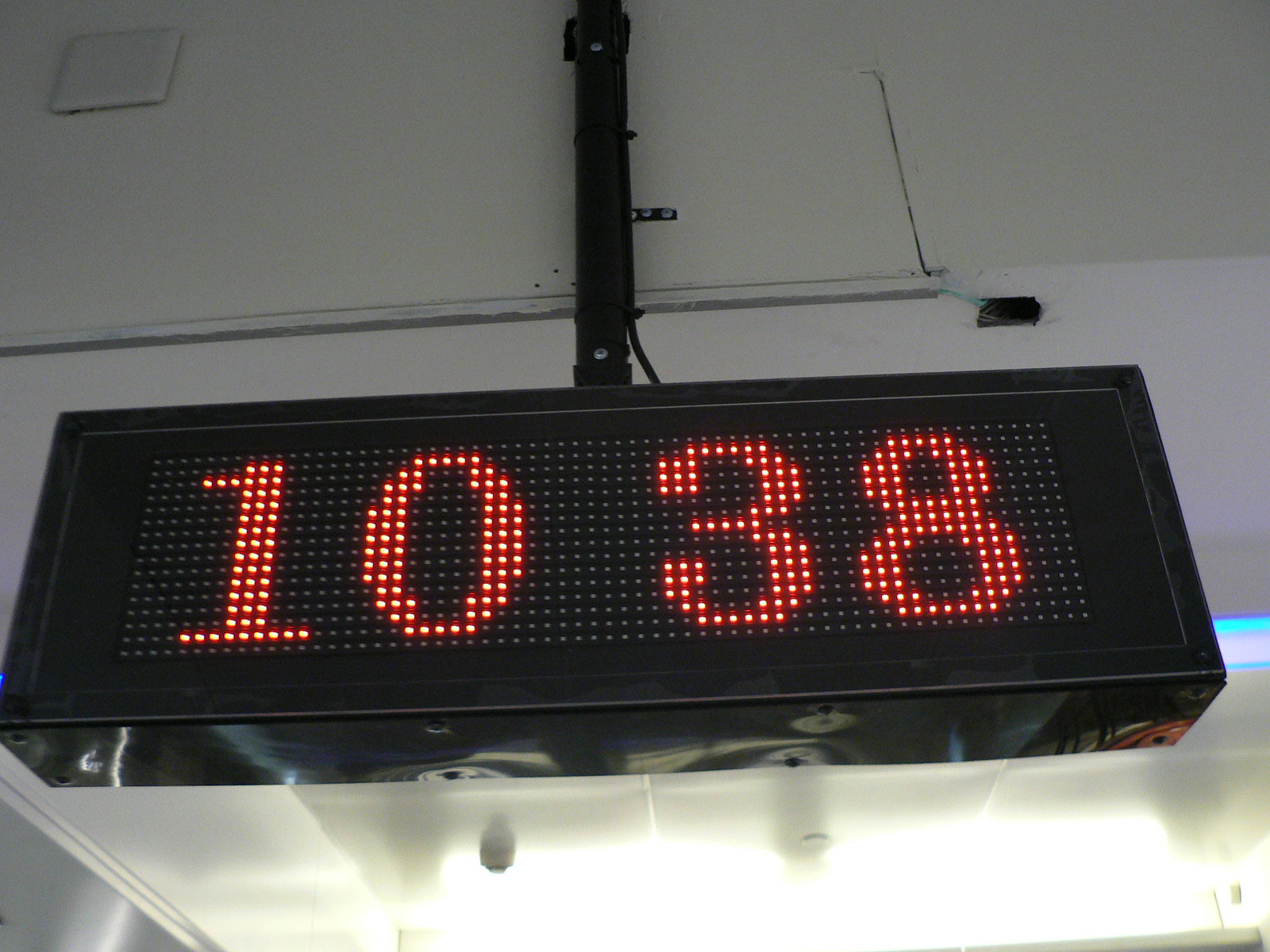The image depicts a digital clock, prominently mounted on a wall. The clock is rectangular with an LCD or LED display that uses a dot matrix to show the time, which reads 10:38. It is connected to the wall by a visible pipe descending from above. The pipe secures the clock in place against what appears to be an overhang or ceiling structure. The clock has a sleek, black, shiny frame that reflects ambient light.

The wall itself is divided into sections by horizontal lines, adding some texture to the background. Below the digital clock, the reflective surface accentuates light reflections. Additionally, the ceiling extends further down in the image, where a very bright light source is visible, casting shadows, glares, and various reflections, adding depth and complexity to the scene.